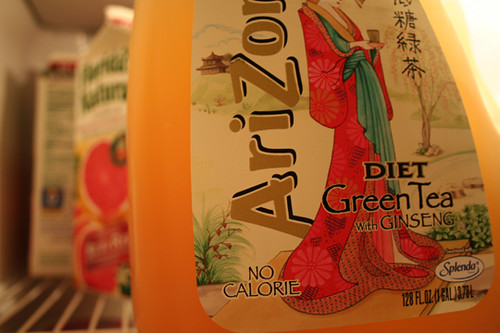This image is a detailed close-up of the lower two-thirds of a plastic gallon jug of Arizona Diet Green Tea with Ginseng, prominently occupying the right side of the frame. The tea jug features a label with the word "Arizona" running vertically up the side and "No calorie" noted beneath it, indicating the use of Splenda as a sweetener. The jug holds 128 ounces (1 gallon or 3.78 liters) of tea. The label is adorned with a depiction of an oriental woman, likely a geisha, wearing a pink robe and green scarf, holding a cup of tea. The background image on the label includes Japanese or Chinese lettering, a traditional house, and surrounding vegetation. 

The left side of the image captures the interior of a refrigerator, with a white horizontal grating at the bottom extending away from the viewer, taking up about 20% of the image's height. Blurred in the background, slightly to the left and partially visible, is a carton of Florida's Natural orange juice, distinguished by an image of a large orange on its label.